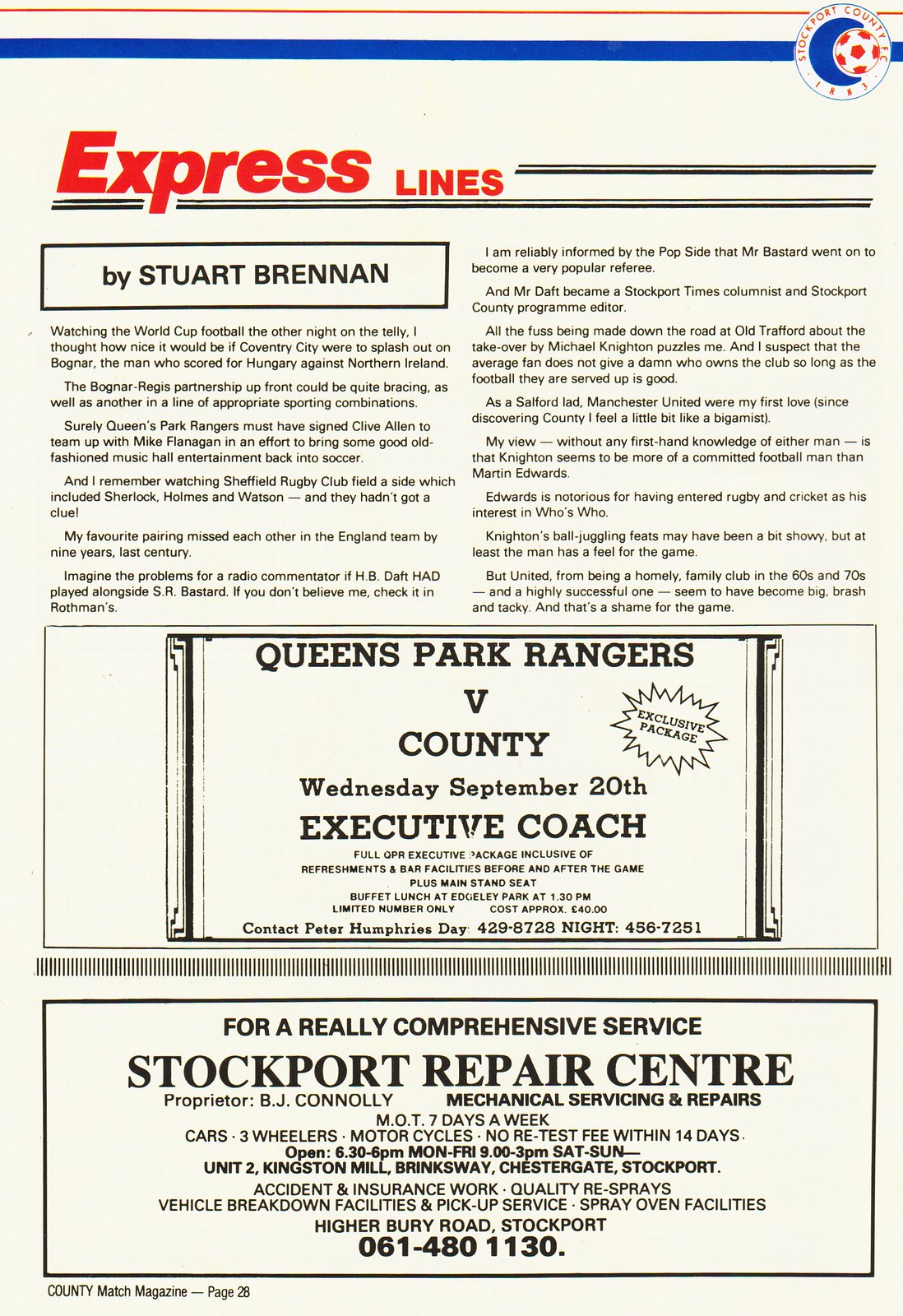This image showcases a promotional flyer for the Express Lines coach service, prominently displaying an article by Stuart Brennan discussing the World Cup soccer. The flyer is in portrait orientation with a clean white background and primarily black text, supplemented with red and blue accents. At the top, a thin red line forms a top border above a thicker blue horizontal line on the right side, featuring a football-themed logo. Directly below, the title "Express Lines" stands out in bold red font. 

The upper portion of the flyer contains a detailed article that not only covers the results and performances of various World Cup teams but also intersperses humorous musings on potential player signings and quirky historical football trivia. Stuart Brennan imagines entertaining combinations like Coventry City signing Bognar, who scored for Hungary, and humorous possible partnerships like HB Daft and SR Bastard from historical England teams.

The lower half of the flyer is dedicated to local advertisements, featuring rectangular blocks of text presenting two distinct businesses in the Stockport area, which is likely a city in the UK. One ad promotes Stock Park Repair Center, emphasizing their comprehensive service. The text in these sections is straightforward, providing practical information, and maintaining the flyer’s consistent black-and-white color scheme, with subtle red highlights.